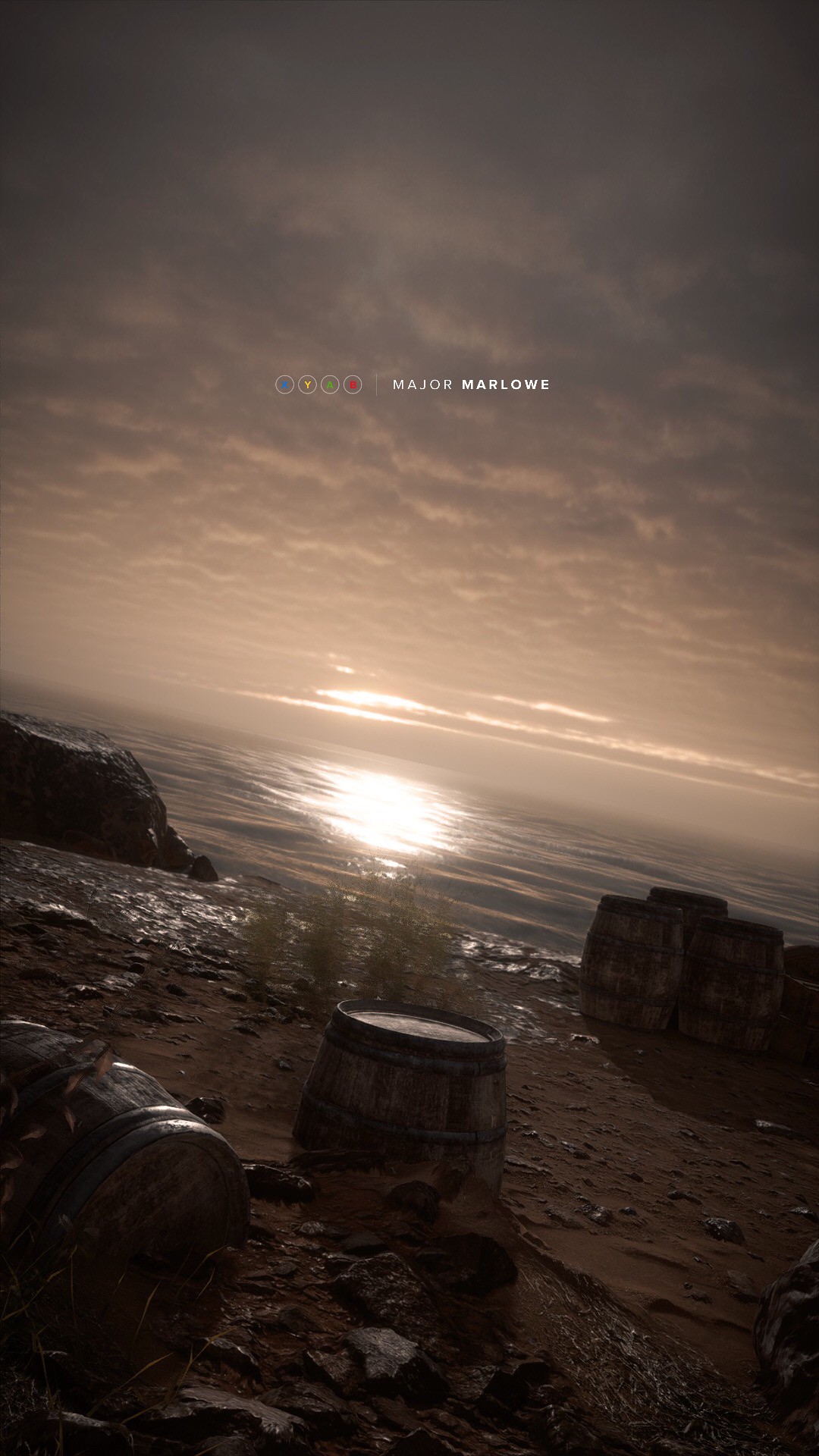In the image, several barrels are situated on the dark, sandy ground at the edge of a body of water. The terrain appears to be a dry patch of land adjoining the water, accentuated by some reflective, possibly wet stone surfaces. A small yellowish plant is sprouting from the soil nearby, adding a touch of life to the scene. There are five barrels in total: a group of three standing barrels rests near the water's edge, one barrel is partially buried in the ground, and a fifth one lies on its side at a distance from the grouped trio. 

The scene is bathed in the warm hues of a bright sunset that reflects off the water, creating a striking contrast with the cloudy sky overhead. In the sky, the words "Major Marlow" are written in white text. Adjacent to this text, there are three small circular icons, which appear to represent letters or controls, possibly for a video game. The icons are color-coded: blue, yellow (with a Y), green (possibly with an A), and red (possibly with a B), hinting at a control scheme for a game.